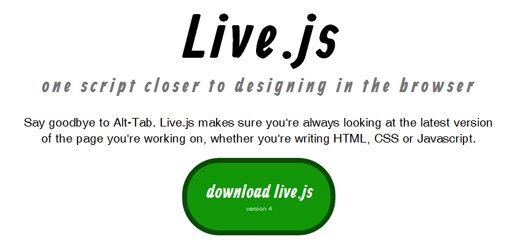This is a screencap of the live.js website, presented on a solid white background. At the top, in prominent dark, bold black lettering, the text "live.js" is displayed. Just beneath this, in slightly smaller, gray font, it reads "one script closer to designing in the browser." Continuing downward, in a different font that is not bold, the caption states: "Say goodbye to alt-tab. Live.js makes sure you're always looking at the latest version of the page you're working on, whether you are writing in HTML, CSS, or JavaScript." This text is all centered within the image. Below this descriptive text, there is a solid green button with a dark hunter green outline. The button features white lettering that reads "Download live.js," matching the font style of the top title. At the bottom of the image, it indicates "version 4."